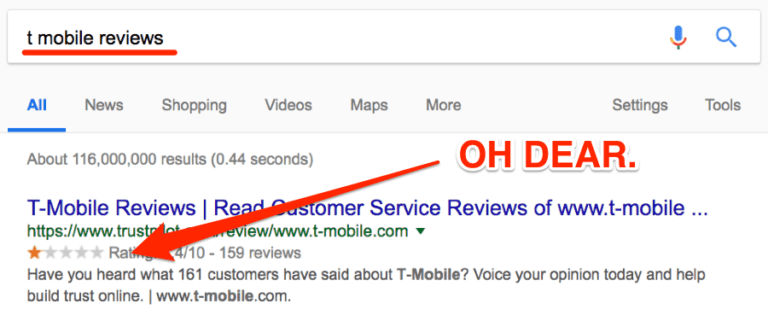In this screenshot, we observe a Google search results page specifically for "T-Mobile reviews." The categories available for further exploration include All, News, Shopping, Videos, Maps, More, Settings, and Tools. Notably, the search produced approximately 116 million results in just 0.44 seconds.

Prominently highlighted in orange is the exclamation "Oh Dear!" which draws attention to the prominently displayed T-Mobile review rating. An arrow points to the review summary, revealing that T-Mobile is rated 1 out of 5 stars, translating to a score of 4 out of 10 based on 159 reviews. A call to action reads: "Have you heard what 161 customers have said about T-Mobile? Voice your opinion today and help build trust online," encouraging users to contribute their own reviews and experiences to help shape collective trust in the service.